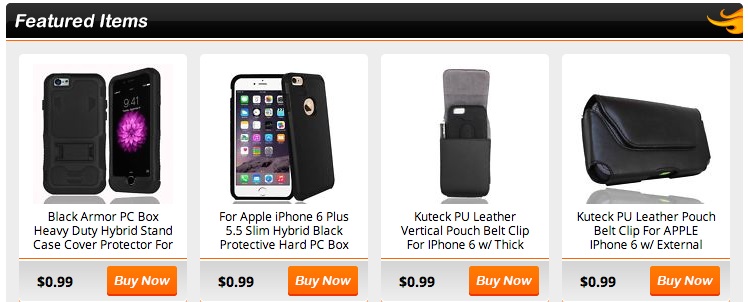The image displays a section of an e-commerce website specializing in electronic items and accessories. At the very top left corner, a black banner prominently features the text "Featured Items" accompanied by a partially visible flame icon. Directly beneath this banner is a thin gold line adding a touch of elegance. The background of the section is in light gray, providing a neutral canvas.

The section showcases four distinct products arranged in a grid format. 

1. The first product is an image of a phone with the description "Black Armor PC Box." It is further detailed as a heavy-duty hybrid stand case, cover protector. Priced at 99 cents, it includes a bold "Buy Now" button in a vibrant red-orange rectangle.

2. Next to it is another phone described for Apple iPhone 6 Plus 5.5. The product is specified as a slim hybrid black protective hard PC box. It is also priced at 99 cents and features a "Buy Now" button.

3. The third item is a KOOTECH PU leather vertical pouch belt clip designed for the iPhone 6 with thick dimensions. This item is advertised at 99 cents with an accompanied "Buy Now" button.

4. The final product in the row is another KOOTECH PU leather pouch belt clip for the Apple iPhone 6, specified for use with external accessories. It, too, is priced at 99 cents and includes a "Buy Now" button.

Each product is clearly labeled with a price and a call-to-action button, emphasizing affordability and prompt purchase options.